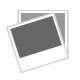This image features a vintage Japanese wooden juice stand, crafted primarily from bamboo or a similar wood. The stand has a distinctive two-part design: the base is a smaller, square-shaped box with cutouts, painted in a faded light blue and yellow pattern, situated on a white floor against a white or light gray background. Rising from this base, there is a larger, shallow tray-like compartment divided into three sections, likely intended for organizing a variety of fruits. The entire structure is topped with thin, U-shaped bamboo handles positioned at the corners of the tray, meeting and tied together at the center, creating a loop for easy covering or carrying. The object is adorned with light pink, white, and subtle gray detailing, adding to its vintage aesthetic, and it's displayed in a well-lit area ensuring all features are clearly visible.